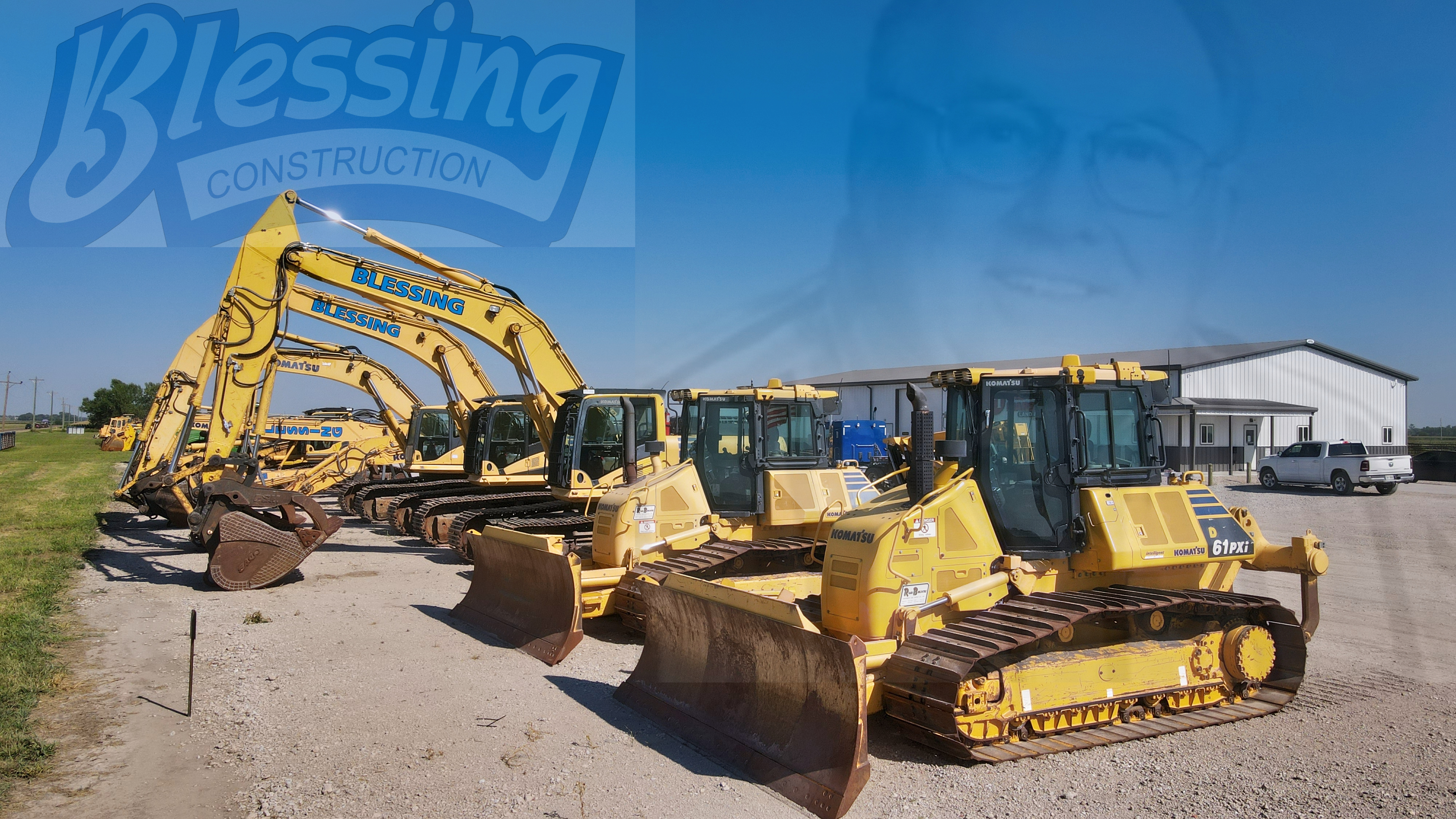The photo, taken outside during the day, features a fleet of large, yellow Caterpillar trucks, specifically loaders and backhoes, arranged in a row on a mostly dirt-covered area. They are equipped with tractor-like treads instead of wheels, allowing them to navigate hilly terrain and assist with various construction tasks such as digging. Some of the machinery has shovels attached, while others are equipped with long cranes and large shovels. The vehicles show signs of rust, indicating frequent use. In the background, to the right, stands a large white building that resembles a warehouse, with a small white four-door truck or an old suburban white car parked nearby. To the left of the frame, there is a patch of grass, but the main focus remains on the heavy machinery. Above the scene, a faded overlay depicts an older man wearing glasses and smiling, likely the owner of the equipment. Beside his image, in the upper left-hand corner, is the company name "Blessing Construction." The photograph suggests a construction company's storage yard and, quite possibly, serves as an advertisement.